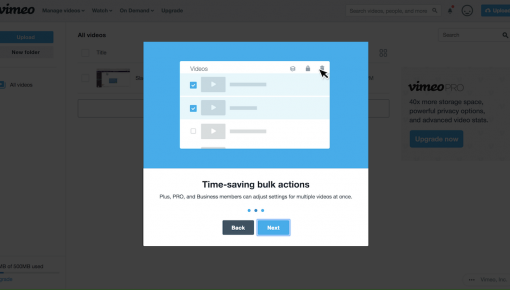The image depicts a web page on a computer screen with a focused pop-up window in the foreground. The background of the main web page is slightly grayed out, drawing attention to the pop-up window. The top section of the pop-up, which spans across in a light royal blue color, prominently displays the text "Videos." In the upper right-hand corner of this section, there are three icons visible. Below this, a black cursor arrow points towards a trash can icon.

Further down, the pop-up contains three small boxes lined up vertically. The top two boxes are checked, resulting in a blue background with a white checkmark in each. Both of these boxes have turned into a light blue color. The third box, however, remains unchecked, maintaining a white background. Despite this, all three boxes include a white play button set against a gray background.

At the bottom of the pop-up, the text "Time-saving bulk actions" is displayed. Flanking this text are two buttons: a black "Back" button on the left and a blue "Next" button on the right. The arrangement and coloration guide the user's focus effectively, emphasizing the options and actions available in the pop-up.